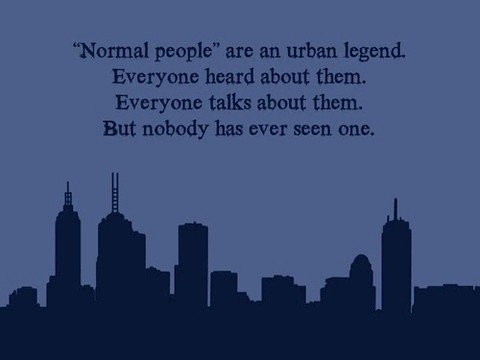The graphic is a minimalist poster featuring the silhouette of a city skyline, possibly New York, against a twilight sky. The skyline at the bottom includes a variety of buildings, with some resembling iconic structures like the Chrysler Building or Empire State Building, and is rendered in a dark blue or navy color. The backdrop of the sky showcases a gradient of dark blue with hints of purple, creating a serene twilight atmosphere. At the top, separated from the cityscape, is a piece of black text that reads, “Normal people are an urban legend. Everyone heard about them, everyone talks about them, but nobody has ever seen one.” This text stands out clearly against the lighter blue tones of the sky, making the message easily readable. The overall design is simple and elegant, emphasizing both the urban landscape and the profound text.